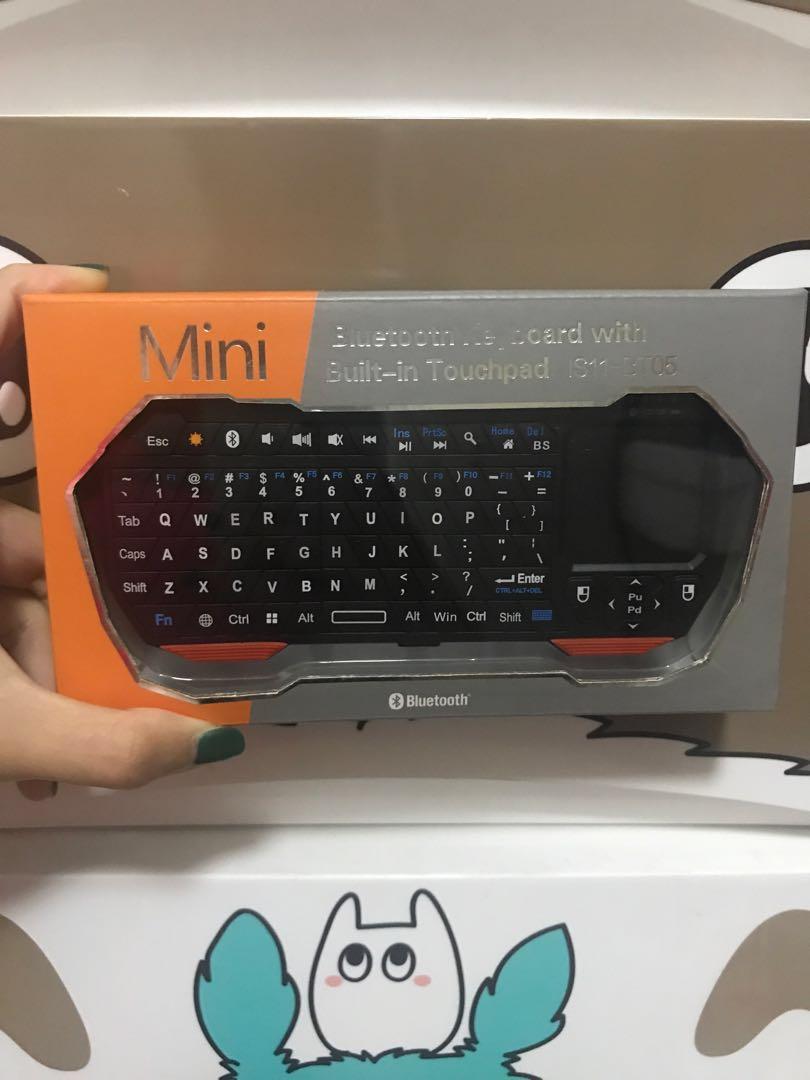The photograph showcases a mini Bluetooth keyboard with a built-in touchpad, held delicately between the thumb and index finger of a hand with dark green painted nails. The keyboard is encased in a box, which is divided into an orange section on the left labeled "mini" and a gray section on the right with the text "Bluetooth keyboard with built-in touchpad" along with a model number. The box features a transparent plastic window, allowing a clear view of the compact black keyboard inside, which includes a touchpad on the right side. The scene is set against a beige background, and the box appears to rest on another box, adorned with a whimsical, cartoonish design of a white bunny-like figure with eyes, cheek blush, and blue arms on either side. The playful illustration adds a touch of charm to the setup.